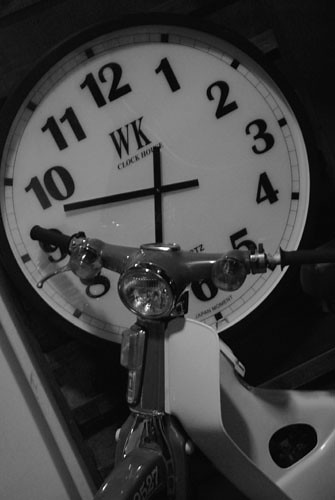This black and white photograph features a vintage scene with a large wall clock and a scooter reminiscent of a Vespa. The clock, with its white face, prominently displays the numbers 1 through 12 in black, with smaller minute markings encircling the perimeter. The clock hands are straight black bars, indicating the time is approximately 9:35. Centrally positioned below the number 12, the clock face bears the bold initials "WK" and beneath them, in smaller lettering, "CLOCK HOUSE." The lower part of the clock is partially obscured, though part of the word "QUARTS" can be faintly made out.

In front of this timepiece stands a small scooter with its handlebars turned away from the clock. While the exact color is indeterminate due to the grayscale nature of the image, the scooter gives an impression of being a dark red with a light-colored backing. The scooter displays various numbers, notably "2527" above the front wheel, and features a black emblem on its white section. This setup evokes an old-time museum exhibit, with the scooter set against a contrasting black resin or plastic frame of the clock. The background shows a white wall leading into darkness, suggesting it might have been taken at night or in a dimly lit space.